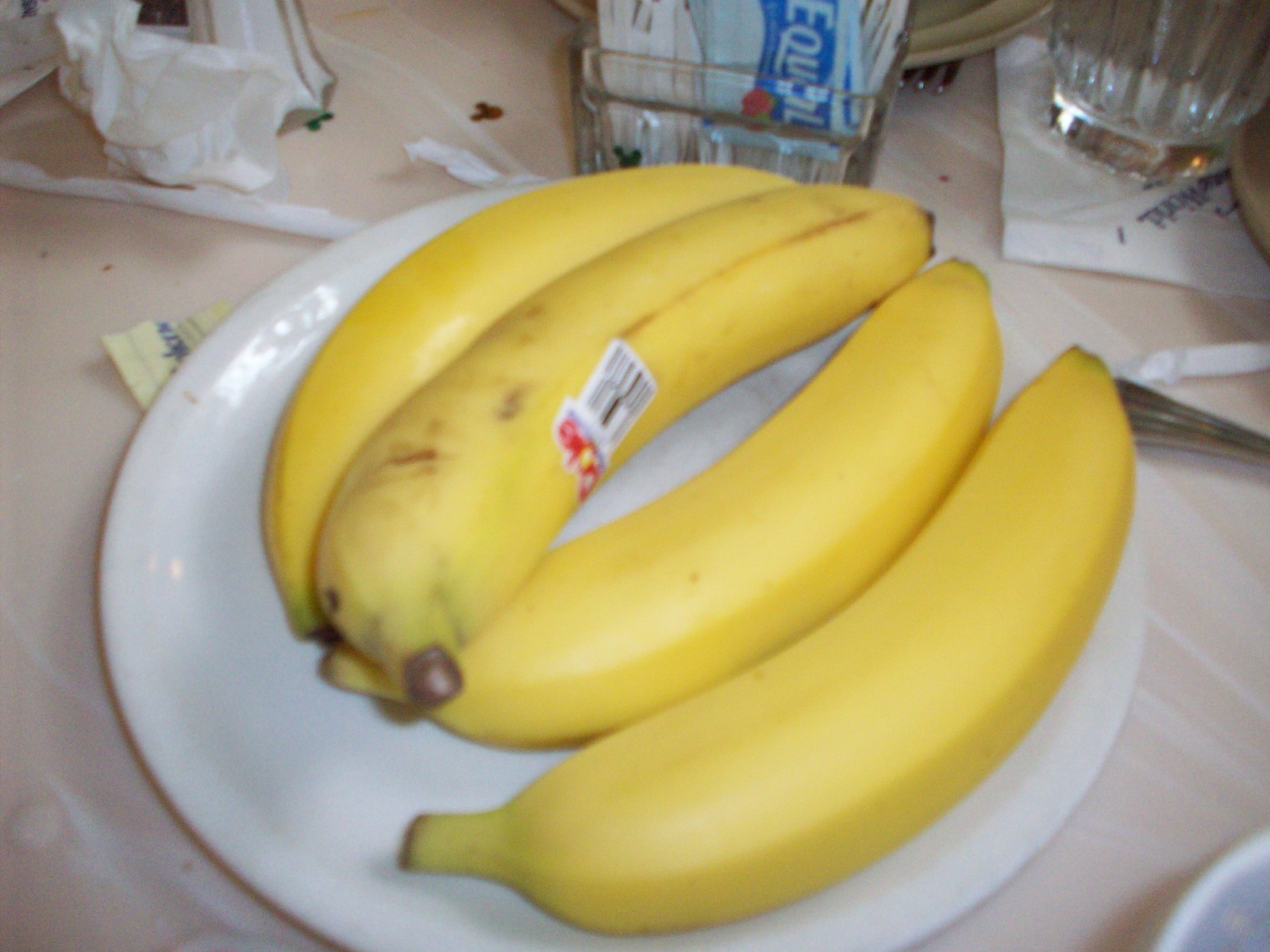In the photograph, the main focus is a cluster of four bananas resting on a pristine white ceramic plate. Notably, the banana positioned in the center bears a small sticker and a barcode, subtly indicating its origin. Captured from a high-angle perspective, the camera looks directly downward, showcasing the bananas as the central subjects, occupying approximately 60% of the frame. The scene is set atop a light cream-colored wooden table, surrounded by a scattered array of common household items that add to the casual, lived-in atmosphere. In the top right corner, a cup can be seen placed on a white napkin adorned with blue text. Adjacent to this setup, there is another plate with the handle of a fork peeking into view. Moving towards the top left, the image captures crumpled tissues and remnants of a paper straw wrapper, contributing to the overall disarray. Despite the surrounding clutter and the slight blur of the bananas, the photograph's composition draws the viewer's eye to the central theme of the image—the humble yet prominent bananas set against their daily backdrop.